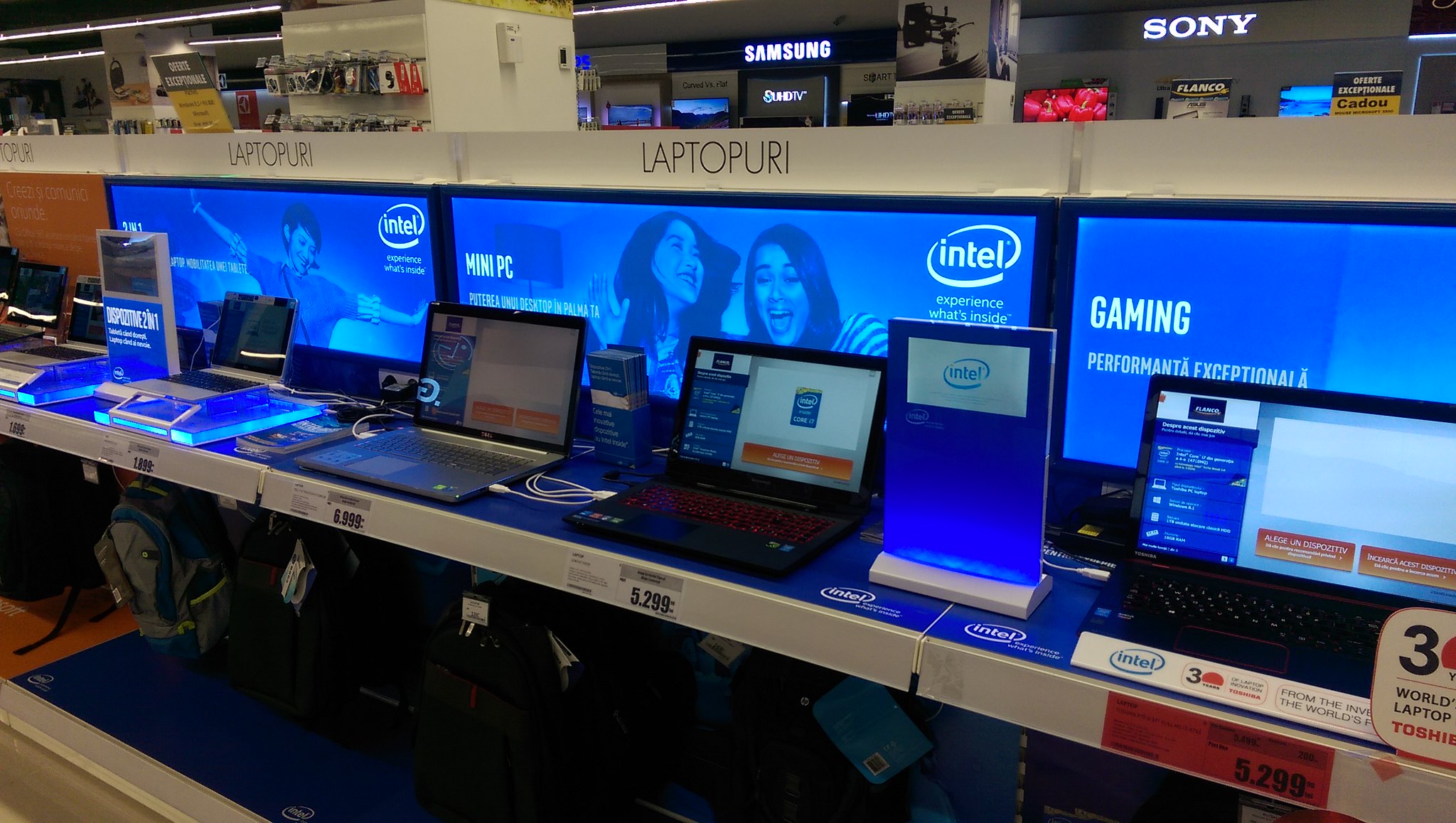This detailed image captures an electronics store's display area, primarily featuring a wide, blue counter showcasing various laptops. At least five laptops, varying in size with the largest on the right, are neatly arranged on the counter. Each laptop is powered on and plugged in with white power cords, allowing customers to interact with the open screens displaying detailed specifications such as RAM and other components.

Prominently, one of the price tags in front of a laptop is marked in orange, listing a price of $5,299, likely in a currency other than US dollars. This particular laptop is an Intel-based Toshiba, noted as the "3 in the world" laptop. Adjacent to this laptop, there's another Intel device, this time a tablet, and another Intel-branded laptop featuring a distinct red keyboard.

In the background, various advertising posters and electronic displays are visible, illuminating brand names like Sony, Samsung, and Intel. These signs also promote different categories such as "gaming" and "mini PC." Notably, there’s a poster including an image of a woman, adding a human element to the technical environment. The overall setting is bright and inviting, designed to draw customers towards exploring and experiencing the latest in computer technology.